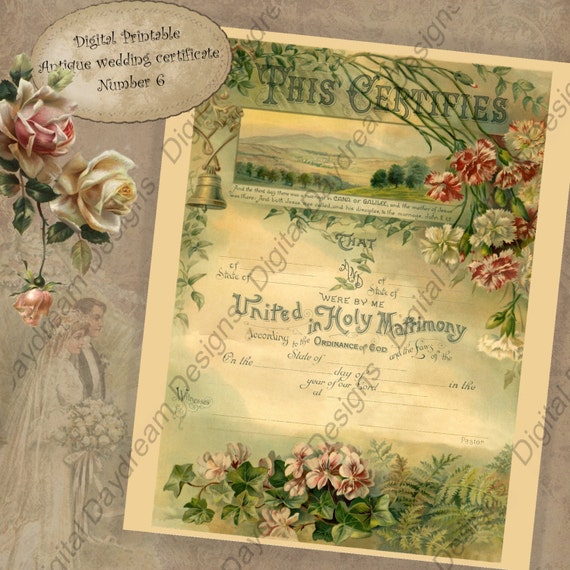The image is a digital illustration of an antique-style wedding certificate titled "Digital Printable Antique Wedding Certificate No. 6." On the right side, the ornately designed certificate features stylized text that reads "This certifies that" at the top, and "United in Holy Matrimony, in accordance to the ordinance of God" in the center. The document includes blank spaces for the names of the couple, as well as fields for the state and date. The certificate is decorated with elaborate floral patterns, including pink and yellow roses with green leaves, and a bell design on the left side. The background of the image depicts a man and woman getting married. Watermarked across the picture is the phrase "Daydream Designs Digital." At the bottom left corner of the image, there is additional text that repeats the title of the certificate.